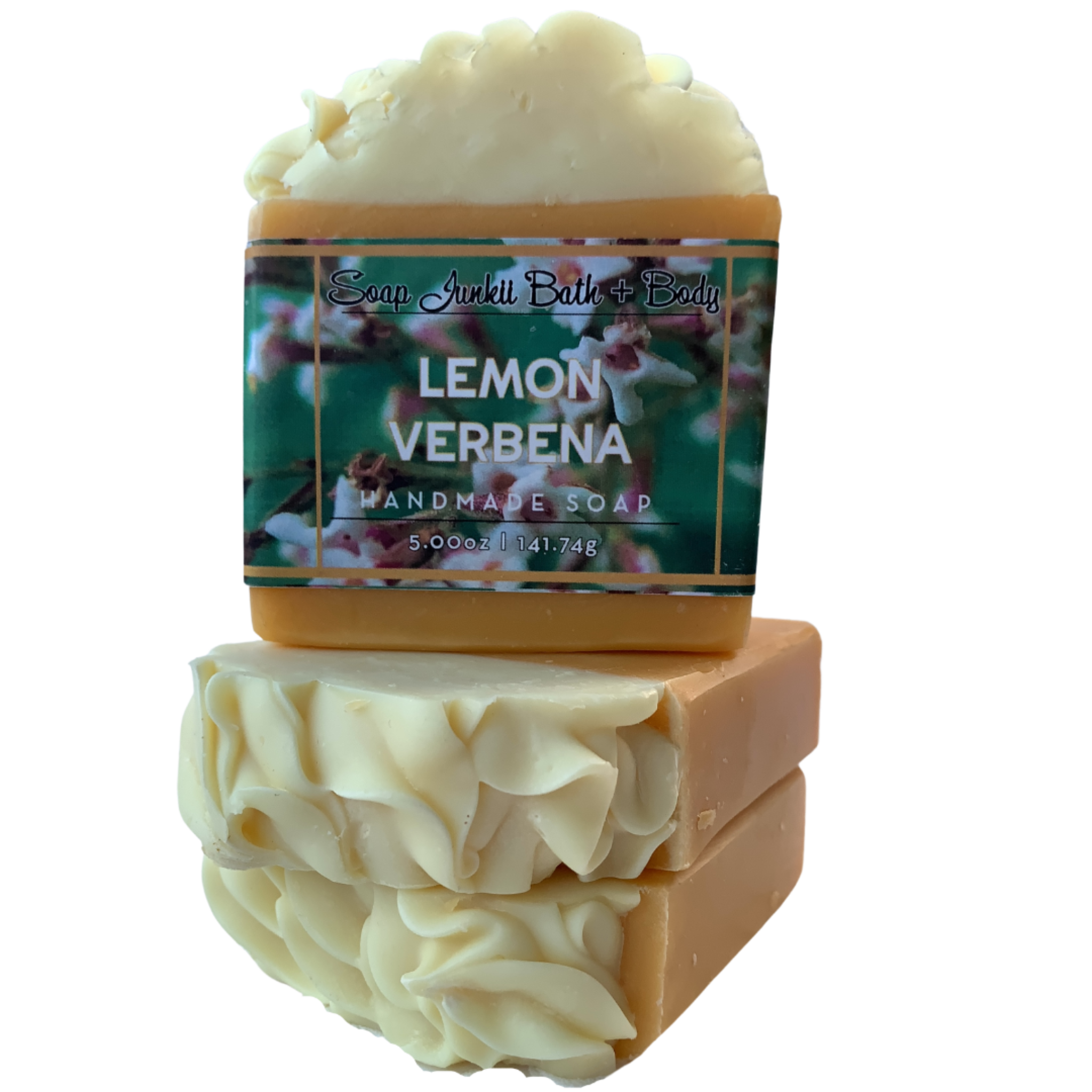The image showcases three handmade bars of soap arranged in a plain white background. Two bars lie at an angle on the bottom, while the third bar stands upright on top of them. These soaps exhibit a gradient from a creamy white top to a orangish-brown base. The upright soap prominently displays a green label featuring a floral background of pink and white buds against green foliage. The label reads "Soap Junkii Bath and Body" in black cursive at the top, "Lemon Verbena Handmade Soap" in white text below, followed by "5.00 oz / 141.74 g." The central focus of the image is on the label and the delicate color gradation of the soap bars.